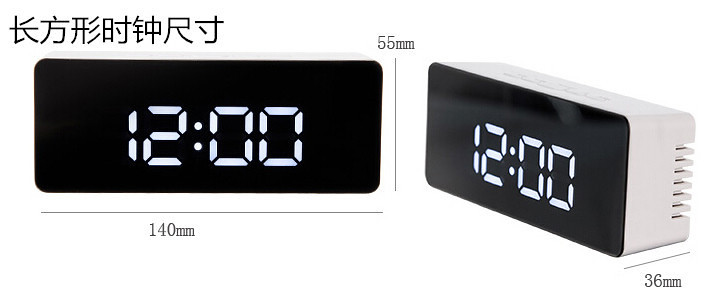An image features a complex arrangement of clocks and measurement symbols. On the left side of the image, there is a clock displaying white text on a black square, indicating the time 12:00. Above this clock, in the top left corner, are various symbols.

On the top right of the image, there is a measurement of "55 milliliters" next to a vertical black line. Extending horizontally from this vertical line is another line marked "140 millimeters." 

The right side of the image showcases another clock positioned diagonally. This clock has a thick white frame surrounding a black face, with the time also shown as 12:00. Below this clock, a measurement reads "36 millimeters."

The diagonally-placed clock features five buttons on its top, enumerated from 1 to 5, suggesting functionality for settings or adjustments. On the right-hand side of this clock, there are a series of divots that create a textured pattern, which would feel like distinct holes if touched.

This intricate composition of clocks, measurements, and symbols suggests a detailed and technical display.